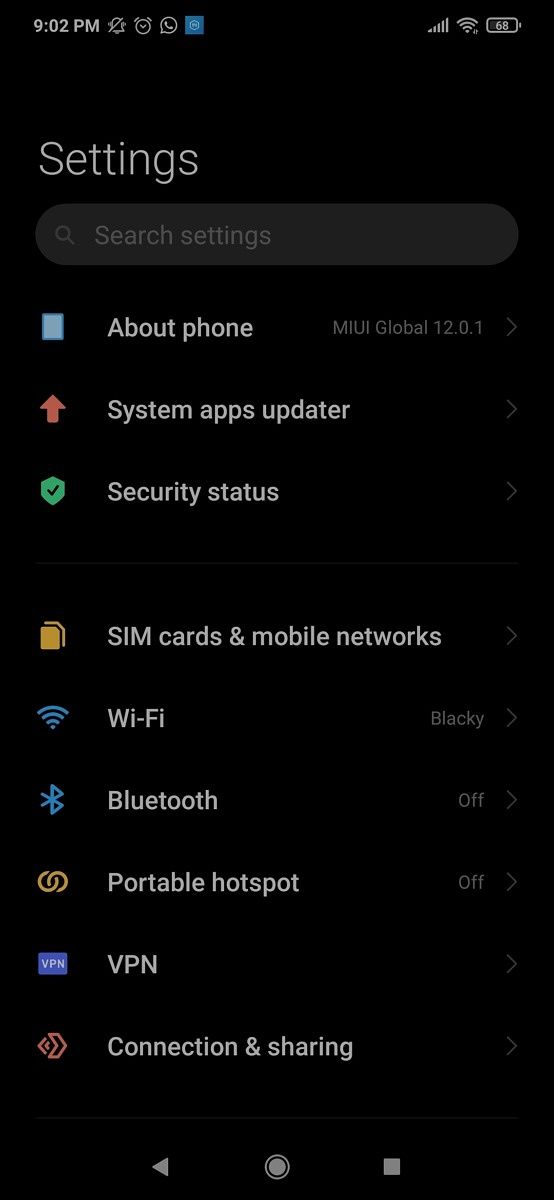This screenshot displays a smartphone set to nighttime mode, evident from the dark background and gray lettering at the top. The time reads 9:02 PM, and the top status bar shows an active alarm, good Wi-Fi reception, and a battery at 68%. The screen is within the "Settings" menu, featuring a search bar labeled "Search settings."

Below the search bar, the first listing is "About phone," accompanied by a blue icon, showing the device runs on "MIUI Global 12.01." Following this are various settings categories: a pink area labeled "System app updater," and an area indicating security status with a VPN logo.

Farther down, a yellow section titled "SIM cards & mobile networks" is visible, along with another section labeled "Wi-Fi," which shows "Blackie" as the connected network. Options for "Bluetooth" and "Portable hotspot" are turned off, each marked with their respective icons. A blue VPN logo appears next to "VPN," which currently has no active connections. Lastly, an orange "Connection & sharing" section is shown but contains no details.

Overall, the setup indicates an organized phone settings menu with various configuration options, some of which are highlighted by color-coded icons.